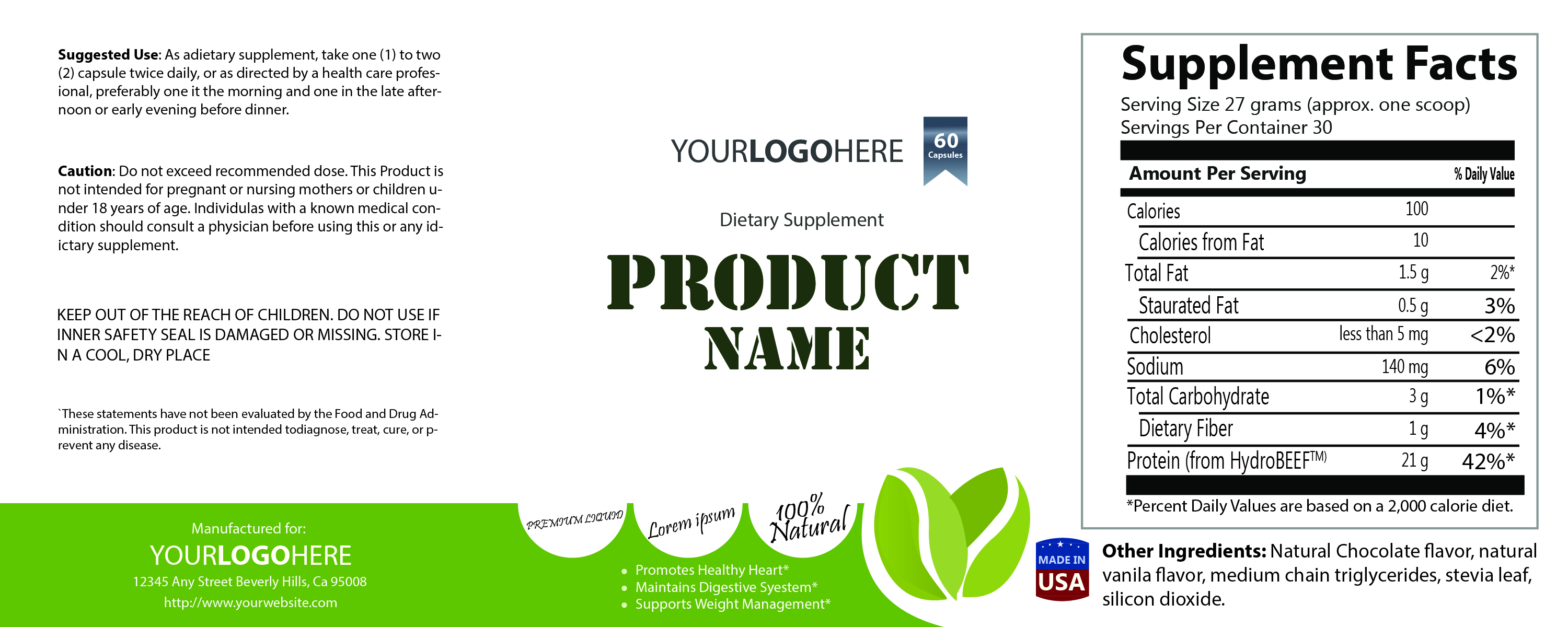This image features a detailed mock-up of a nutritional product label designed for customization. The left side of the label, set against a white background, includes three small paragraphs in black text that outline suggested use, caution instructions, and a warning to keep out of the reach of children. The bottom of the label features a green banner stretching across the entire width, except beneath the ingredient panel on the right. This banner contains the text "Your Logo Here" and incorporates a scalloped design with wave-like curves and leafy illustrations.

At the center of the label, also on a white background, it states "Your Logo Here" in black, followed by "Dietary Supplement Product Name" in blue beneath it, set inside a ribbon shape. The right side of the label presents the supplement facts within a white square bordered in black. This section details the serving size of 27 grams (approximately one scoop) and the number of servings per container (30). It lists various nutritional components including 100 calories, 10 calories from fat, 15 grams of total fat, 65 grams of saturated fat, less than 5 milligrams of cholesterol, 100 milligrams of sodium, 3 grams of total carbohydrates, 1 gram of dietary fiber, and 21 grams of protein derived from hydro beef. The bottom of the right panel also contains the ingredient list and a blue and red "Made in the USA" stamp resembling a barrel. 

Overall, the label is a well-organized, customizable template ideal for various dietary supplement products, with clear sections for branding, usage instructions, nutritional information, and additional product details.